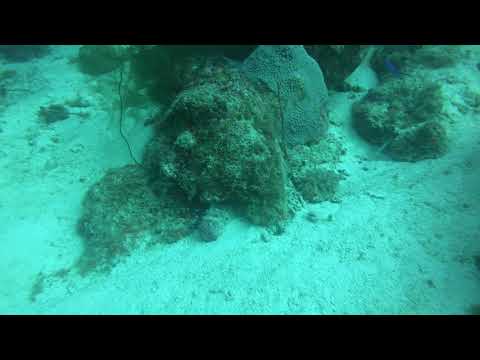The photograph captures an underwater scene depicting the seafloor of a body of water. The image is framed by rectangular black bars at the top and bottom. Predominantly displaying a low-resolution, murky aqua green atmosphere, the seafloor consists primarily of white, rocky sand. Central to the image is a cluster of plant-like formations, appearing tan and green, with porous, leafy qualities. Surrounding these formations are various brown tendrils, contributing to their rock-like appearance. Additional similar formations are visible in the distance, giving a sense of depth. The scene appears desolate, with no fish or other marine life present, and the overall ambiance is serene and somewhat eerie.